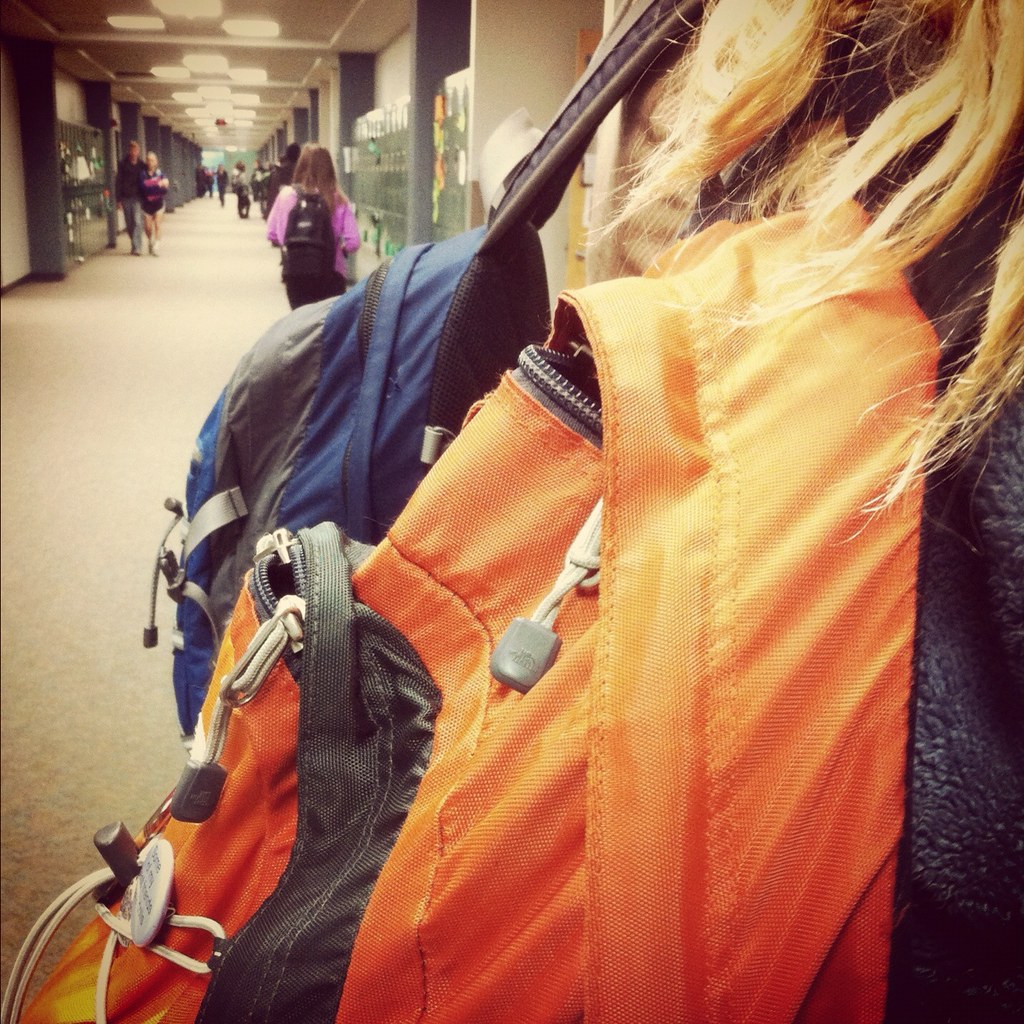The photograph captures a bustling school hallway with white carpeting. Looking down the hallway, several people are seen walking. The main focus is on a person in the bottom right-hand corner, who has long blonde hair, possibly with brown highlights, flowing down their back. They are wearing an orange canvas backpack with two zipper pouches, both slightly open, revealing signs of wear. To the left of the orange backpack, they are carrying a second backpack, which is blue with a black strap. In the distant background, there are dark green lockers on both sides of the hallway, and various other students walking by. One girl in a pink sweater with a black backpack stands out. Near a glass display case on the left side of the image, a possible parent and child can be glimpsed, suggesting a lively school environment, perhaps a high school or middle school.